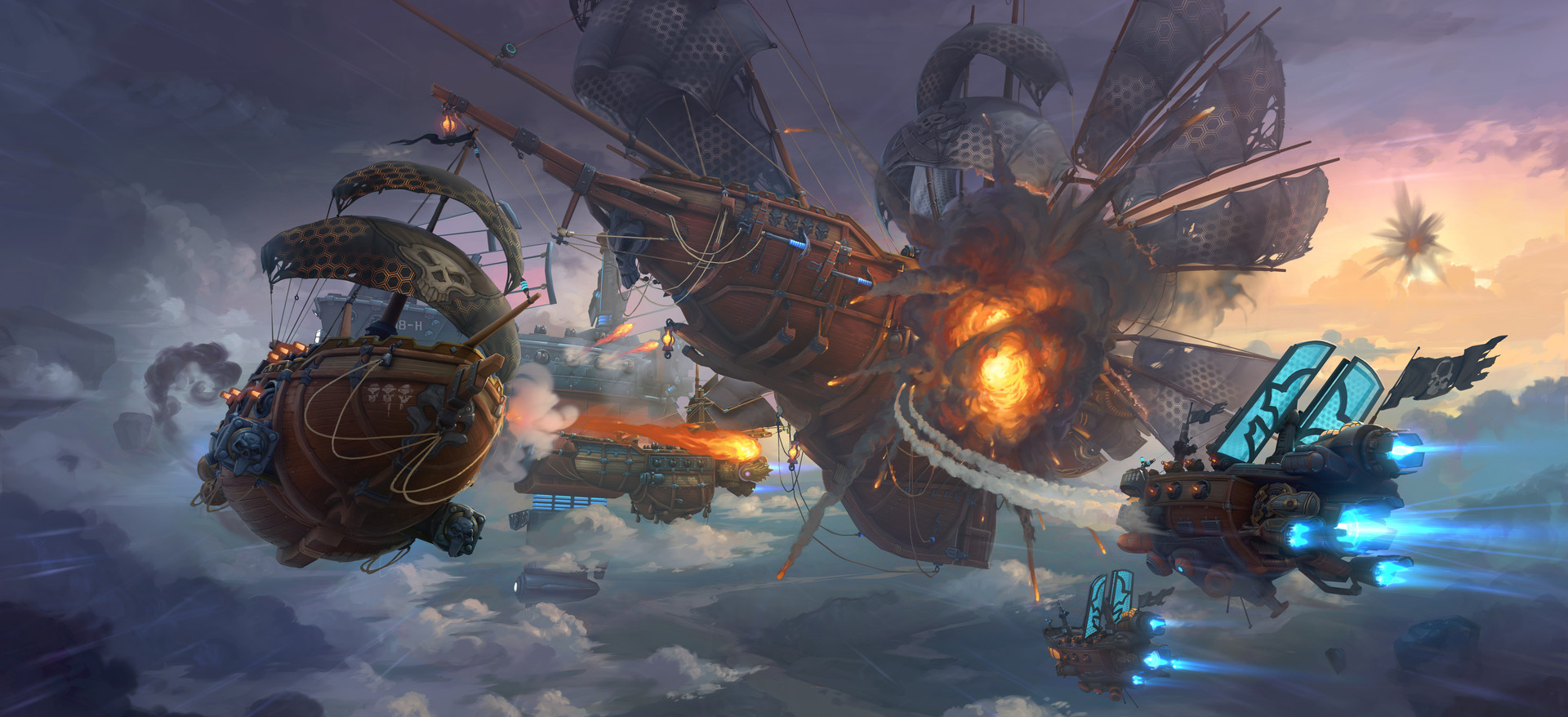The image is a highly detailed 3D graphic rendering depicting an intense aerial battle scene between flying steampunk ships and smaller, high-tech fighter crafts. Central to the scene is a large, damaged steampunk ship, ablaze and billowing smoke from being struck by missiles. This ship, adorned with sails protruding at various angles and mesh-covered sections supported by poles and cables, exhibits a mix of old-timey and modern elements, including metallic structures and advanced weaponry. Surrounding this main ship are other airborne vessels engaged in combat, some resembling pirate ships with skull insignias on their sails. The sky is filled with clouds, with the sun partially obscured in the distance on the far right. Additional smaller ships, equipped with jet engines emitting blue flames, navigate through the chaotic scene, firing upon the larger vessels. The entire tableau suggests a sci-fi, steampunk battle high above the ground, blending historical aesthetics with futuristic technology.